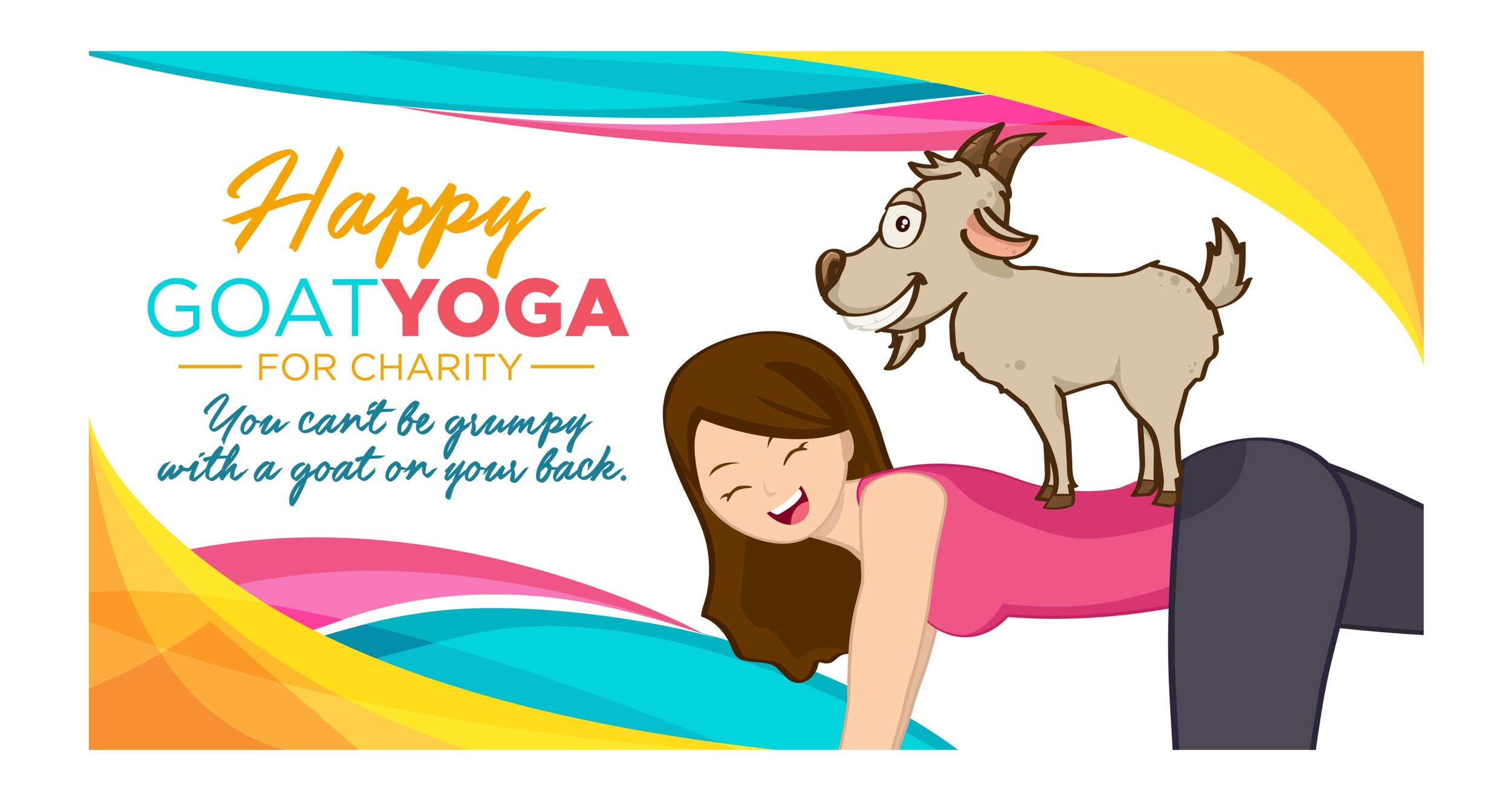This vibrant, colorful flyer advertises "Happy Goat Yoga for Charity" and features an energetic and playful design. The top right and bottom left corners showcase swirling gradients of orange, yellow, teal, and hot pink, adding a cheerful and dynamic border to the flyer. These swirly motifs are echoed across the entire piece, providing a lively, whimsical backdrop. In coordinating colors, the main text reads, "Happy Goat Yoga," with "for Charity" right below it, all in bright, bold fonts. The catchy tagline, "You can't be grumpy with a goat on your back," appears in a dark teal script, adding a touch of elegance.

Central to the flyer is a cartoon illustration of a joyous young woman with brown hair, dressed in a pink sleeveless shirt and black yoga pants. Positioned on her hands and knees in a yoga pose, she is happily laughing and looking towards the viewer. A sweet, smiling light brown goat with dark brown horns and blue eyes stands playfully on her back, reinforcing the fun and unique nature of the yoga event. The overall design, with its colorful swirls and cheerful imagery, captures a sense of joy and community, enticing viewers to join in the fun for a good cause.